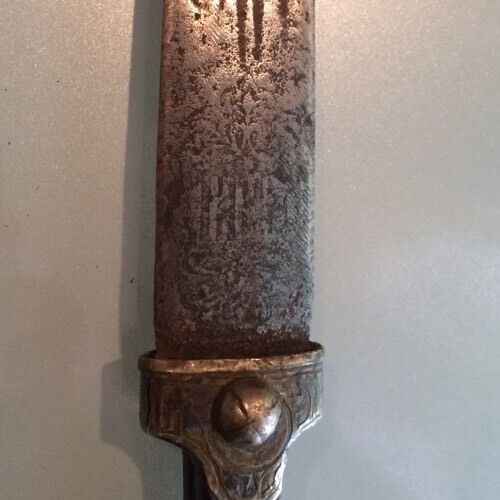This is a detailed close-up photograph of the mid-section of what appears to be an ancient, possibly medieval Norseman's sword, mounted against a plain, shiny white or light grey background, emitting a dull, soft glow. The image reveals the blade and part of the hilt, highlighting the heavy weathering and the patina accumulated over centuries, which has left the metal tarnished and rusty. The sword's blade shows remnants of faded inscriptions and intricate designs, now nearly obliterated by time. The T-shaped hilt, likely made of bronze, features a round bolt embellishment in the middle, which has small divots and resembles an ancient type of fastening mechanism. This bolt appears to bind the blade to the handle, suggesting a craftsmanship that involves detailed metalwork perhaps from the 1400s to the 1700s. The sword's surface also displays numerous scratches and indentations indicative of its age. The lighting from above creates reflections on the blade and casts a shadow to the left, enhancing the textured, rustic appearance of this historically valuable artifact, possibly displayed in a museum.